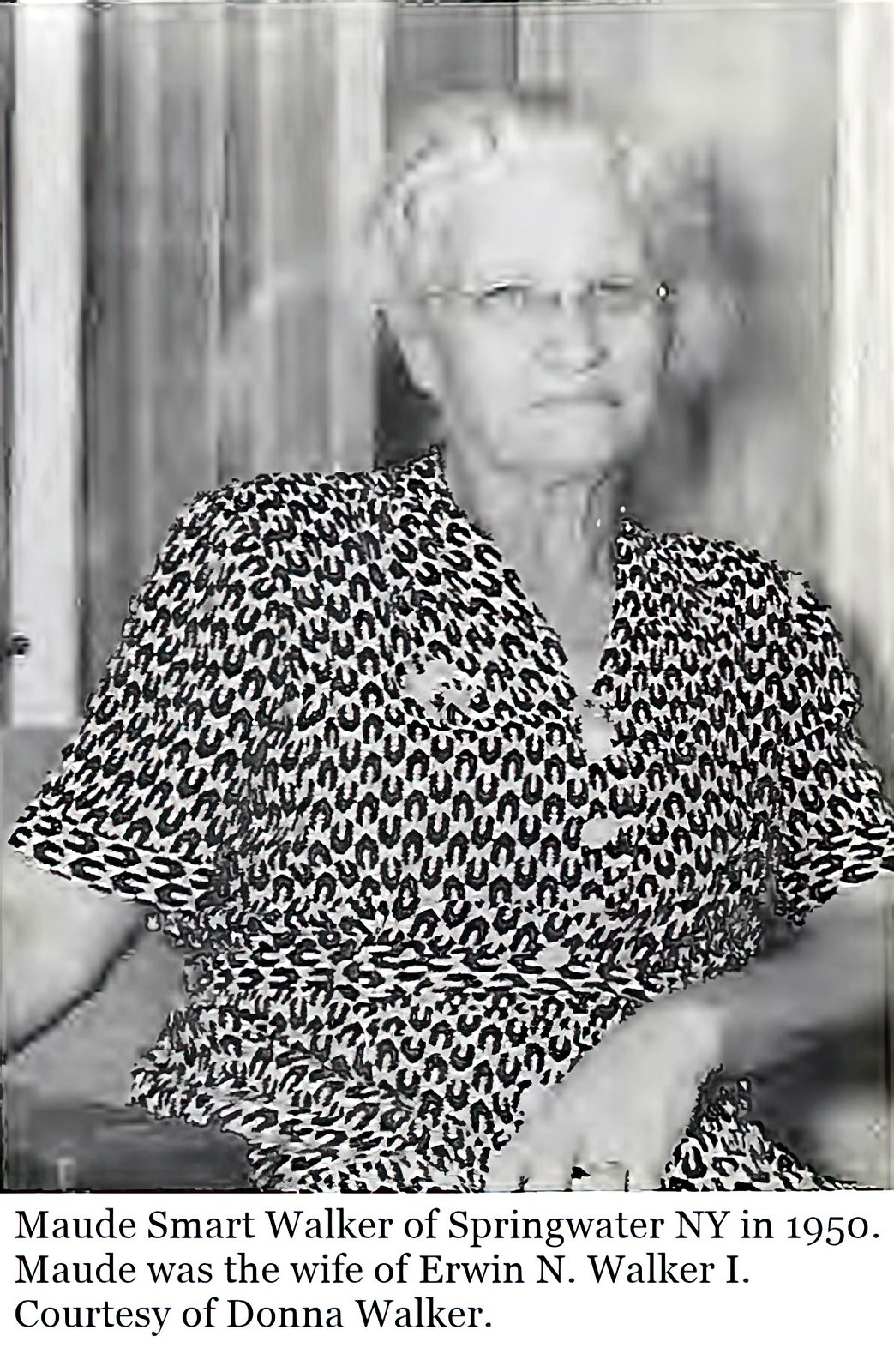This black-and-white photograph from 1950 captures Maud Smart Walker of Springwater, New York. Maud, the wife of Erwin N. Walker I, courtesy of Donna Walker, is seated, wearing glasses and a patterned short-sleeved dress with buttons down the front. Her white hair is neatly pulled back, and she wears a neutral expression on her face, not quite smiling nor frowning. The image is somewhat blurry, particularly around her face and the indistinct background, possibly depicting a wall or drapes, adding to the photograph’s vintage ambiance. Despite the overall blur, the dress appears more defined, creating an intriguing contrast in this portrait of Maud.